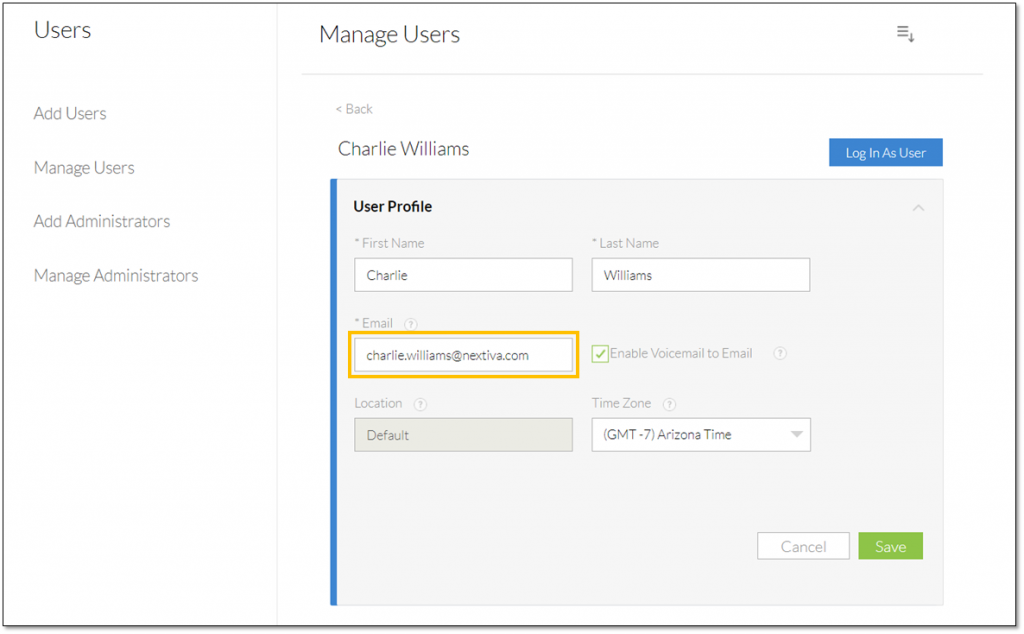The interface displayed in the image features a white box with a gray border and detailed, structured content predominantly in various shades of gray. In the upper left corner, the gray text reads "Users." On the left-hand side, a column lists options in lighter gray text: "Add Users," "Manage Users," "Add Administrators," and "Manage Administrators," separated by a very light gray horizontal line.

To the right, slightly left of center, the section is labeled "Manage Users." On the right side of this section, there is an icon with three dots and a downward arrow. Below that, a gray horizontal bar stretches across the interface.

Underneath this bar, there is a blue button labeled "Back." Below this button, the name "Charlie Williams" appears in blue text. On the right-hand side, a blue button with white text says "Log In as User."

A blue vertical bar runs down the left side of a gray interior box, within which is the black text "User Profile." Inside this section, gray labels for "First Name" and "Last Name" are followed by corresponding text boxes containing "Charlie Williams" in black text. Below that, the label "Email," also in gray, is circled in yellow, with the email address "charlie.williams@company.com" displayed.

Additionally, there is a gray checkbox labeled "Enable Voicemail to Email" that is checked. The "Location" is set to "Default," and the "Time Zone" is indicated as "GMT-7 / Arizona Time." At the bottom left of the image, there are two buttons: a white "Cancel" button and a green "Save" button.